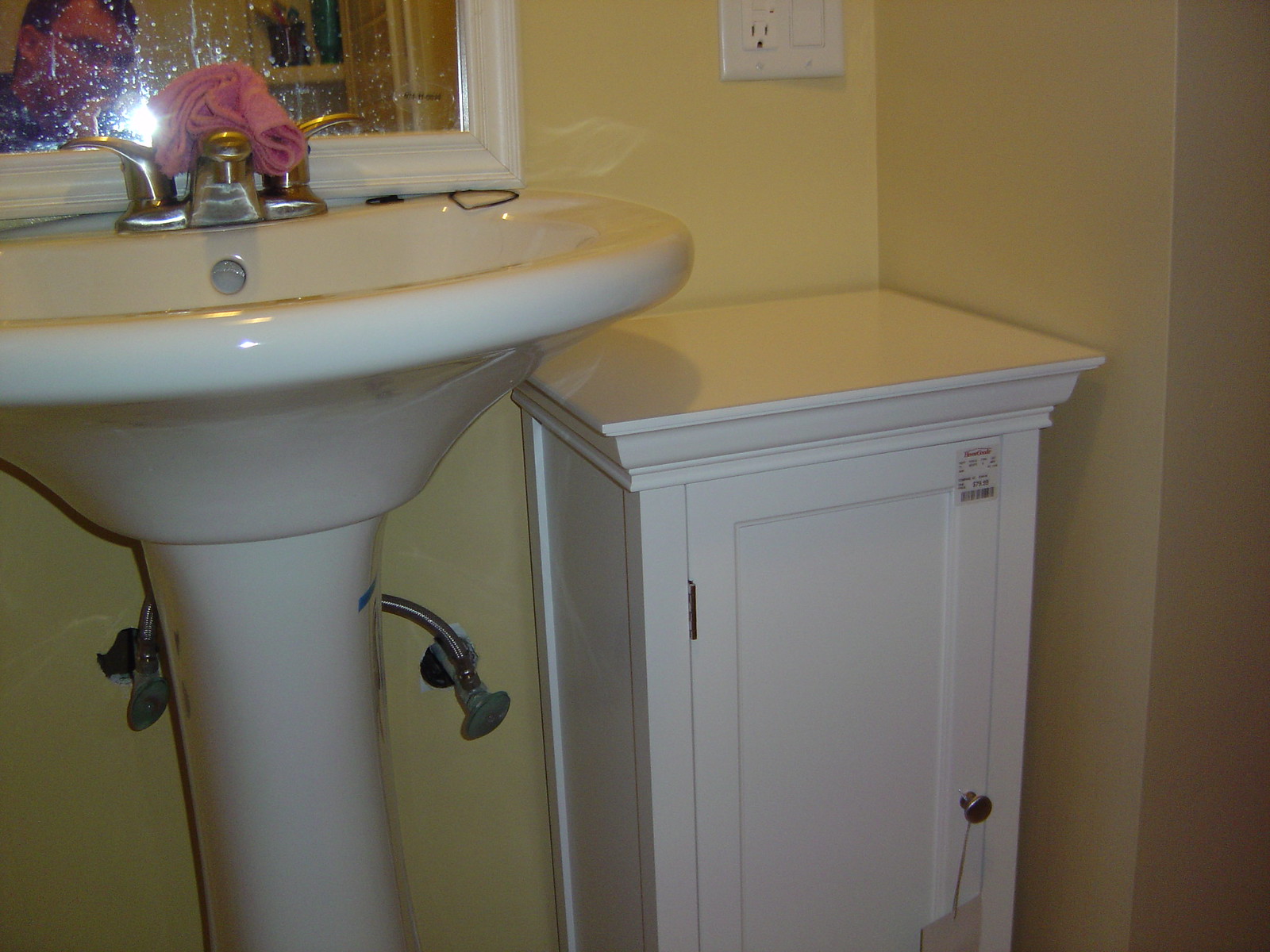A dimly lit bathroom houses a porcelain pedestal sink with an oval basin and no counter space, featuring gold or silver fixtures and adorned with a pink washcloth draped over the faucet. To the sink's right in the corner stands a white-painted cabinet, slightly shorter than the sink, sporting a metal knob and a noticeable white price tag sticker on its top. The pale cream-colored walls host a white light switch with an outlet positioned above the cabinet. A rectangular mirror with a white frame hangs behind the sink, its surface marred by dirt, reflecting a man's head and the illumination from the camera.